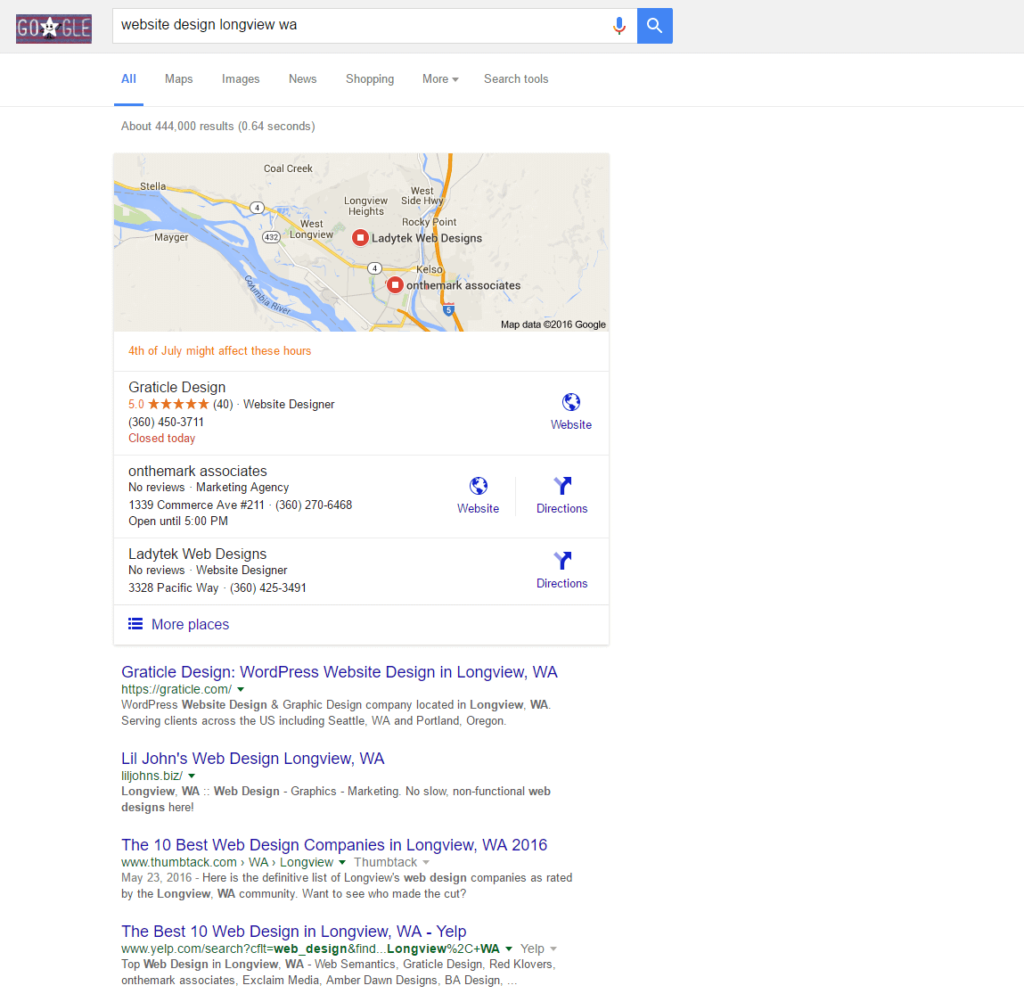**Descriptive Caption for the Image:**

The image displays a Google search results page for the query "website design Longview, Washington." In the top left corner, there's a distinctive Google logo encased in a purple rectangle, where one of the 'O's is stylized as a star. The central search bar shows the entered query, flanked by a microphone icon on the right and a blue square containing a magnifying glass symbol. 

Just below the search bar, the user interface offers clickable options: "All" (highlighted in blue and underlined), "Maps," "Images," "News," "Shopping," "More," and "Search tools." The "All" tab is selected, presenting comprehensive search results. A small gray text beneath states there are approximately 444,000 search results generated in 0.64 seconds.

The main content starts with a Google map pinpointing relevant locations in Longview, Washington. Beneath the map, there are three prominent local search results, each detailing business names, addresses, phone numbers, and additional information options. There’s also a link labeled "More places" in purple for expanded results.

Further down, four website search results are displayed. The first result is highlighted in purple as "Gradical Design, WordPress Website Design in Longview, Washington," followed by a URL and more descriptive information. The second result features "Little John's Web Design in Longview, Washington,” accompanied by additional details and a web address. The third result introduces a list titled "The Ten Best Web Design Companies in Longview, Washington 2016," with a corresponding URL. The final result reads "The Best Ten Web Design in Longview, Washington, Yelp," also accompanied by a web address and further information.